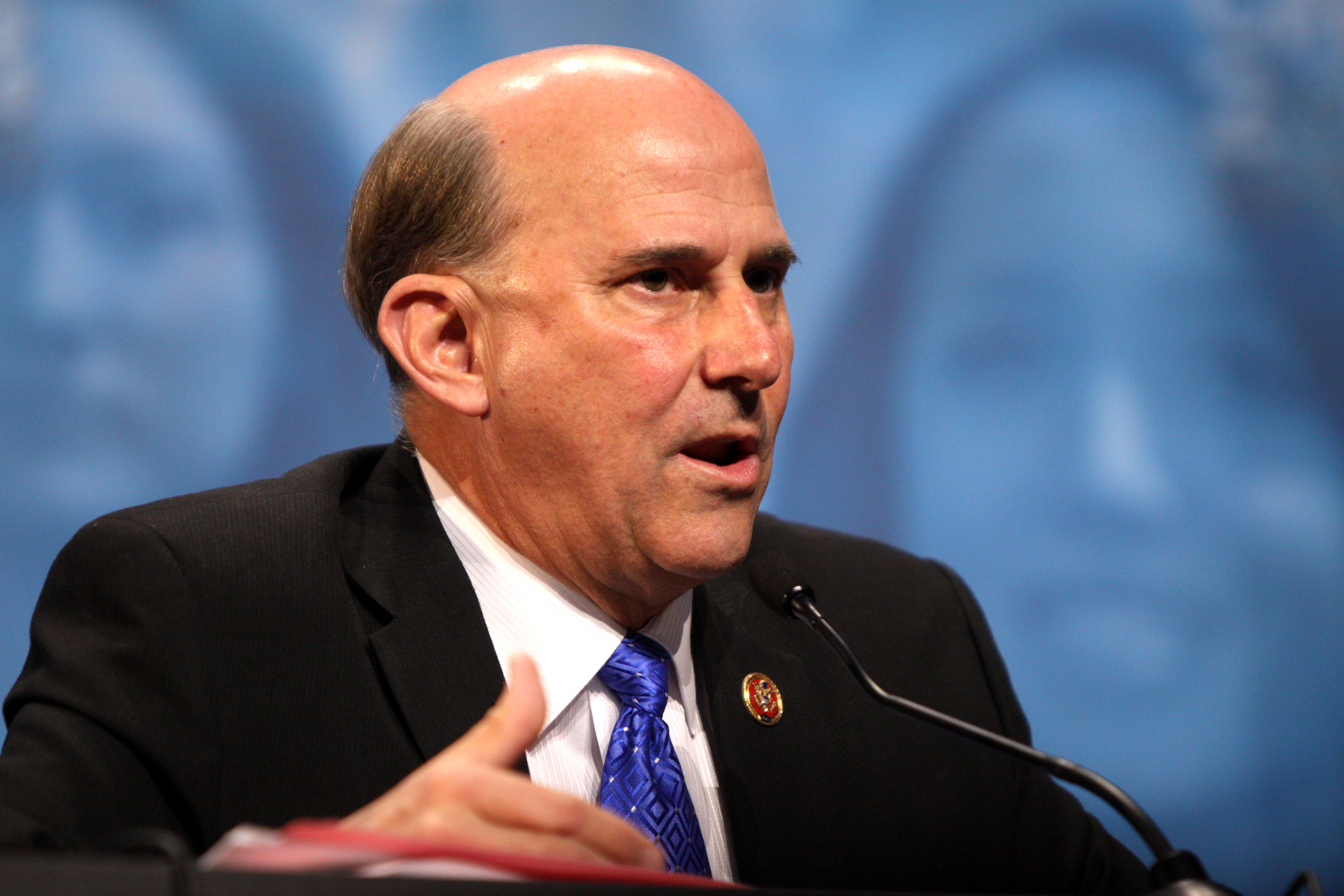In this image, we see a man at the center, speaking passionately into a black microphone positioned at the bottom right of the frame. His mouth is open, suggesting he is speaking intensely. He is balding but has dark hair on the sides, and he is dressed formally in a black suit jacket, a white shirt, and a blue tie featuring a pattern of concentric diamond shapes. An oval pin, colored red and gold, adorns his lapel. His hand rests on a stack of red and white papers or a folder, with his thumb up. The background is blurred, making it difficult to discern details, but it appears to show some wallpaper with faces, possibly women's faces, filtered in blue. The setting seems to be indoors, likely at a press conference. The overall color palette includes blue, light blue, tan, brown, black, gray, purple, and orange, creating a detailed and vivid scene.